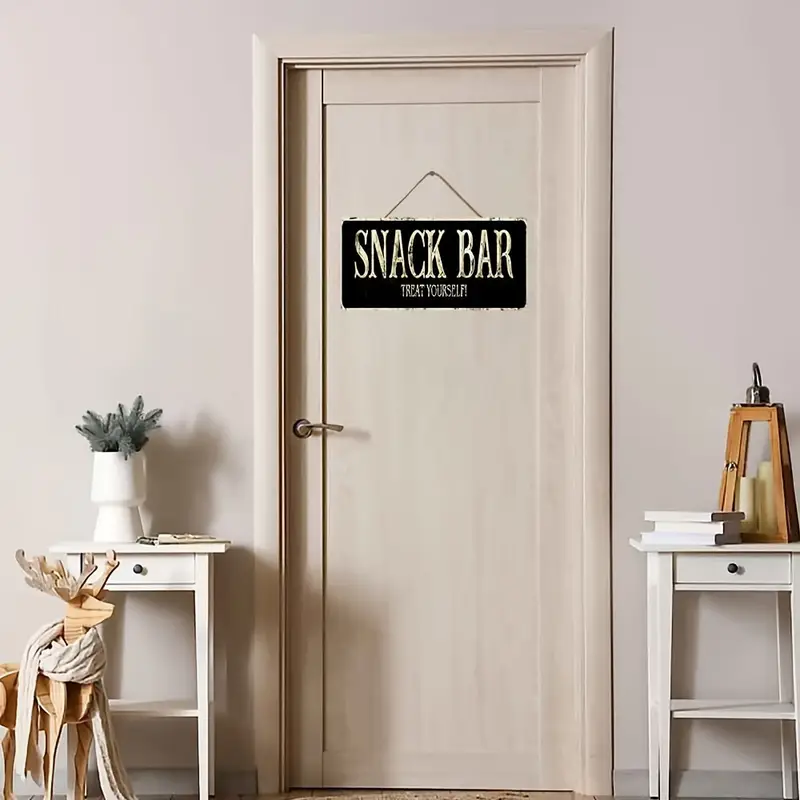This is a square indoor image featuring a closed door that is slightly off-center to the right, flanked by light gray walls. The door is a typical off-white or cream color, bordered by thin wooden panels. It has a curved silver handle positioned on the left side in the center. Hanging on the door is a sign with a black background that reads "Snack Bar" and "Treat Yourself." On each side of the door, there are small white wooden end tables with black circular knobs on their drawers. The left table displays a white vase containing a cactus-like, prickly plant. There is also a tan wooden deer adorned with a scarf to the left of this table. The right table supports a stack of books and two candles on a wooden apparatus. This indoor setting resembles a hallway or living room.